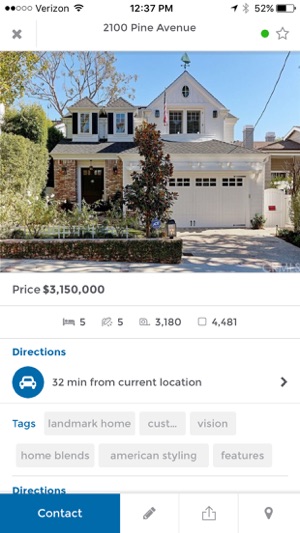This screenshot, captured on an iPhone, clearly displays the familiar iPhone interface elements such as the service provider and Wi-Fi icons on the upper left, the time (12:37 PM) in the center, and the battery and Bluetooth icons on the upper right. The background of the image is predominantly white, indicating that it is taken from a real estate app or website. 

At the top of the screen, just below the time, the listing's address is prominently displayed. The app's primary font colors are white, black, and grey, with notable blue accents. Specifically, two words appear in blue font, accompanied by a blue button labeled "Contact," and a blue circular icon featuring a car, which provides directions to the listing's location from the user's current position.

Beneath the prominently displayed address, there is a picture of the house for sale. Directly below this image, essential details about the property are provided, including the price, the number of bedrooms and bathrooms, and the total square footage. Additional features such as directions and tags are also included in this section.

At the bottom of the screen, the "Contact" button is clearly visible, alongside several other navigational buttons. This organized layout ensures that all pertinent information is easily accessible, offering a comprehensive view of the property listing.